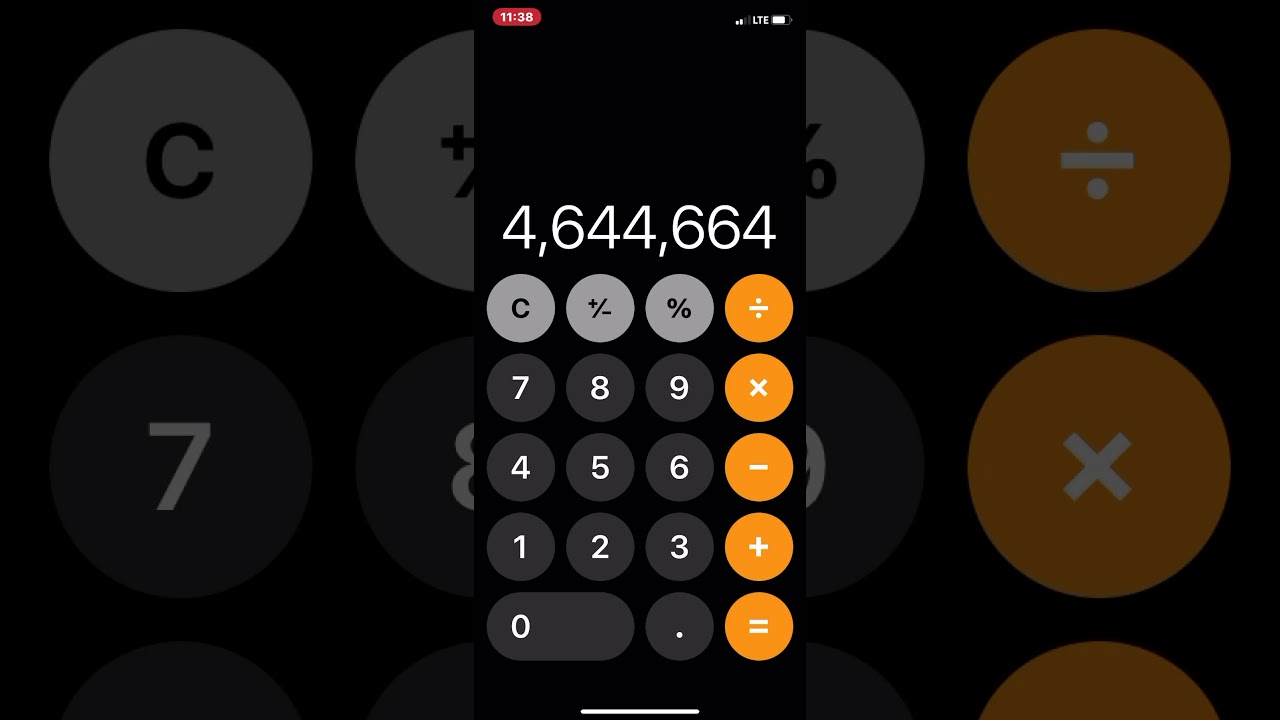In the image, a large black rectangular surface is adorned with various circles and buttons. On the top left, there is a white circle featuring a "C," followed by a gray circle with a white number "7" below it. Adjacent to these, you'll find a white plus-minus symbol and a white percent sign. Further along, there's a gray button with a white number "8" and two yellow buttons, one with a division symbol and the other with a multiplication symbol.

At the center of the black rectangle, there appears to be a rectangular phone screen. The upper left corner of the screen is highlighted in red and displays the number "1138." On the right side of the screen, a nearly full battery icon is visible. The phone's screen shows a calculator application open, with the number "4,644,644" displayed prominently.

Below the display, a series of calculator buttons are arranged in rows. The top row features buttons for "Clear," plus-minus, percent, and division. The second row contains buttons for numbers "7," "8," "9," and multiplication. The third row displays numbers "4," "5," "6," and subtraction. The fourth row includes numbers "1," "2," "3," and addition. The final row features a "0," a decimal point, and an equals sign. The buttons for "C," plus-minus, and percent are gray, while the number keys are black. The buttons for division, multiplication, subtraction, addition, and equals are orange.